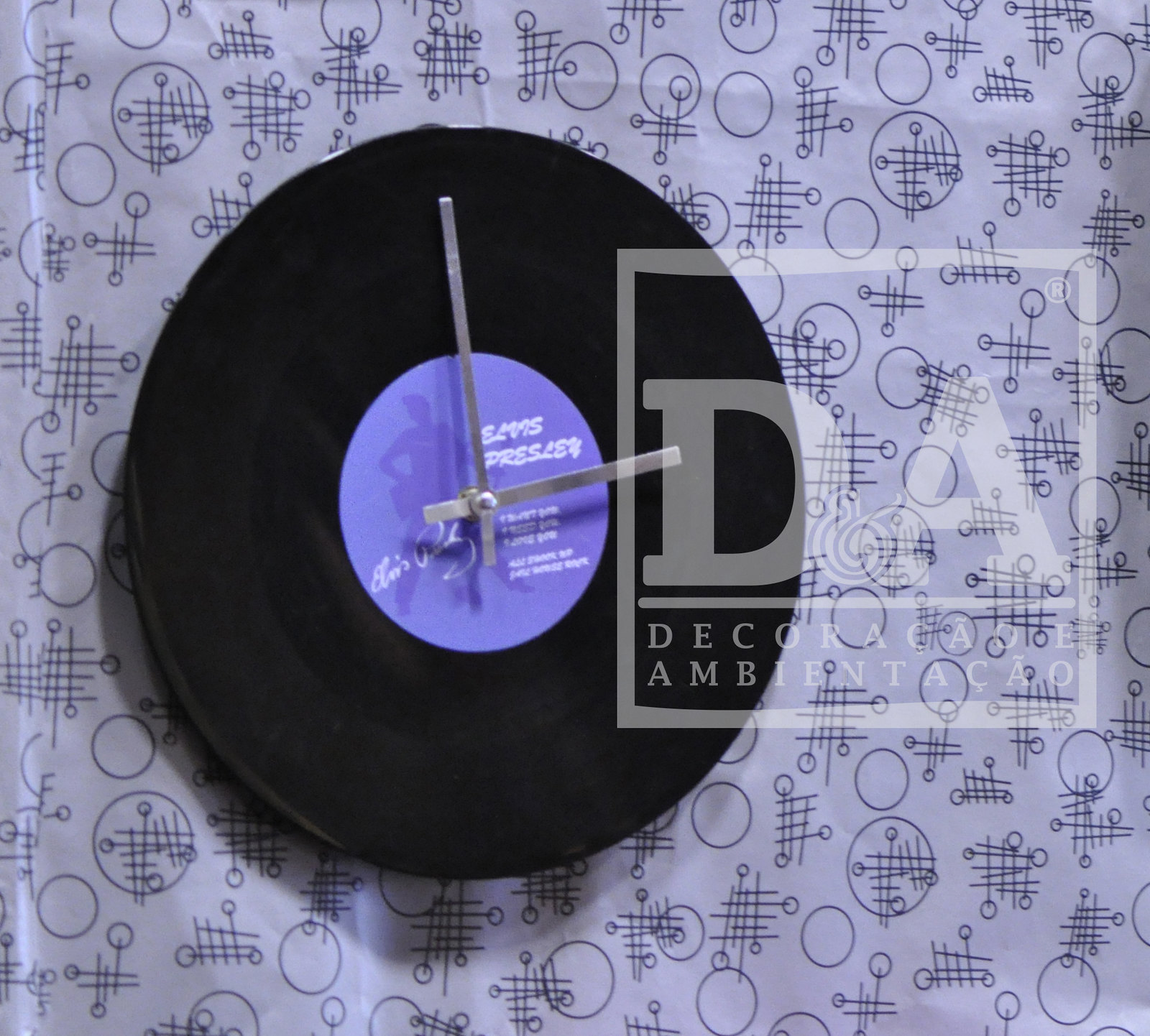The image depicts a distinctive modern clock crafted from a black LP record. At the center of the clock is a lilac label, featuring a white signature that reads "Elvis Presley" and a subtle gray silhouette of Elvis holding his guitar and singing. The clock has silver hands, one long and one shorter, standing out against the dark backdrop of the record. This piece hangs on a wall adorned with an eccentric, geometric wallpaper of light lavender, accented by intersecting circles and lines in blue. Additionally, there's an overlay watermark with large gray letters "DA" and the words "Decoracao Ambientoc" beneath, indicative of a foreign language related to decorations.